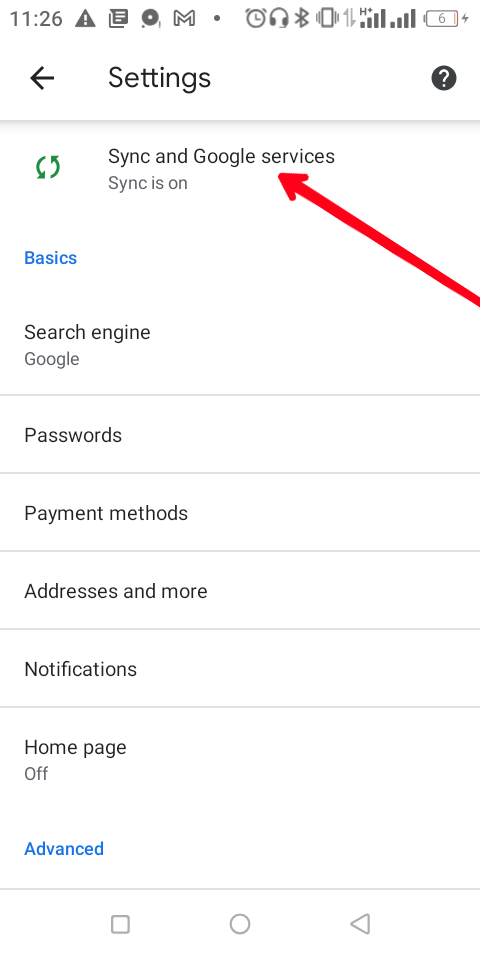The image shows the settings page of a cell phone. At the top center, there is a red arrow pointing towards the word "SYNC" within the Google Services section. The word "SYNC" is displayed in black font, and directly below it, there is the text "SYNC is on." Accompanying this text, you can see the SYNC symbol, which consists of two bent arrows forming a circular shape.

Beneath the Google Services section, the word "BASICS" is written in blue, smaller font. The section below "BASICS" features a vertical list of settings items. The first item on the list is "Search Engine," followed by "Google." The subsequent items are "Passwords," "Payment Methods," "Addresses and More," and "Notifications." Further down, it says "Homepage," which is currently set to "off." At the bottom of the list, the word "Advanced" is highlighted in blue.

In the upper left-hand corner of the screen, the time is displayed, showing 11:26.